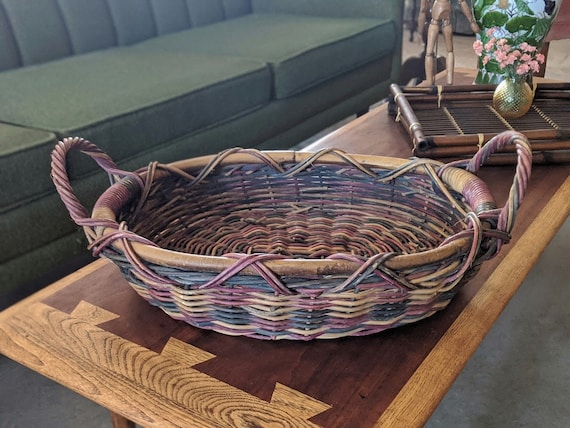The image captures a wicker basket resting on a wooden end table, which features a light wood border with a darker brown center. This table is placed adjacent to a long, green fabric couch. The basket, empty and adorned with two prominent handles, sits towards the left side of the table. The woven wicker pattern is detailed and intricate. Behind the table, there is a flat, square object with two layers, upon which a glass vase filled with pink flowers is placed. The background reveals additional furniture and a grayish carpet, suggesting a cozy seating area. The setting's color palette includes green, brown, and hints of pink and purple, creating a warm and inviting atmosphere.